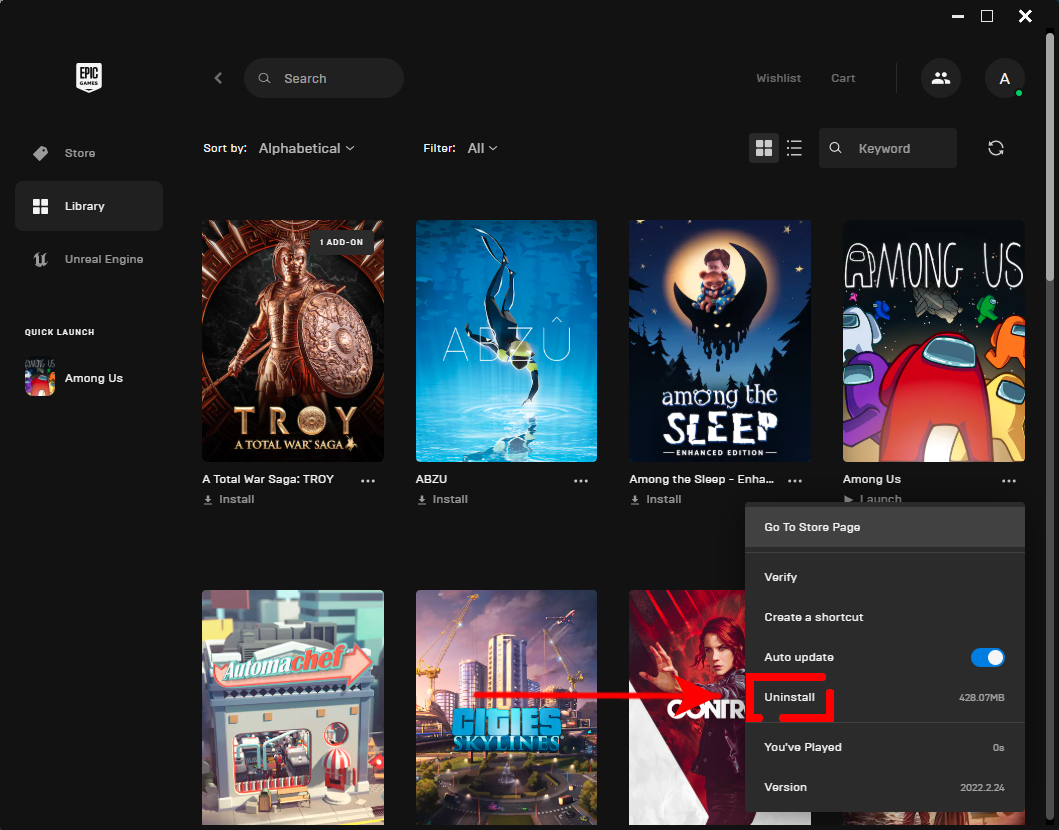Screenshot of Epic Games Launcher Tutoring with Visual Highlights

This screenshot depicts a tutorial interface within the Epic Games Launcher program. The overall color scheme features a black background, white text, dark grey pop-ups, and accent colors.

On the left side, there is a very narrow vertical menu with the Epic Games logo prominently displayed at the top left. Below the logo, there are three key sections with icons on their left for ease of identification: Store, Library, and Unreal Engine. Beneath these sections, a bold text label reading "Quick Launch" is displayed, with "Among Us" currently selected for quick launching. The cover image of "Among Us" appears to the left of its title.

To the right, the screen displays the main content area, the game library. This section maintains the same dark color scheme but organizes the content into two rows and four columns of game covers. Each game cover includes its title and specific icons indicating their availability status, such as "Launch" or "Install."

A dark grey pop-up in the game library highlights the uninstallation process, with critical areas circled and a red arrow along with a line prominently indicating the "Uninstall" option. The visual aid clearly outlines the steps necessary to remove a game from the program.